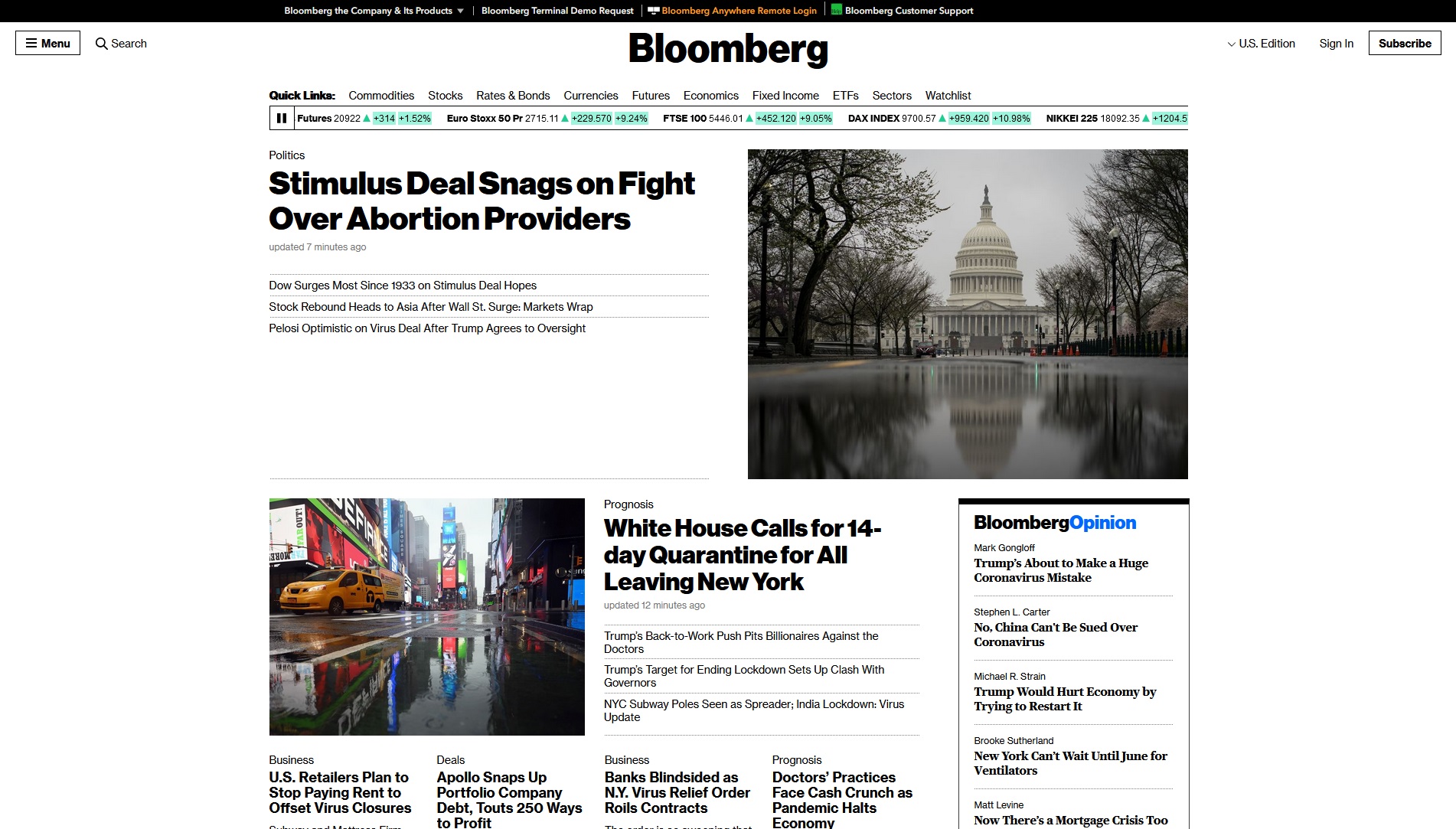The image features a black border along the top, with text that is too small to be read clearly. Set against a white background, the prominent headline reads "Bloomberg," followed by various section headers including "Quick Links," "Commodities," "Bonds," "Currencies," "Futures," "Economics," "Fixed Income," "ETFs," "Sectors," and "Watch Lists." 

Underneath these sections, there is a category named "Politics" with a headline that states "Stimulus Deals Snag on Fight Over Abortion Providers." To the right, the image shows a picture of the U.S. Congress building surrounded by trees. Below this image, there is a picture of Times Square in New York with accompanying headlines: "Prognosis: White House Calls for 14 Day Quarantine for All Leaving New York," "Trump's Back to Work Push Pits Billionaires Against Doctors," "Trump's Target for Ending Lockdown Sets Up Clash with Governors," "NYC Subway Seen as Virus Spreader," and "India Lockdown: Virus Update."